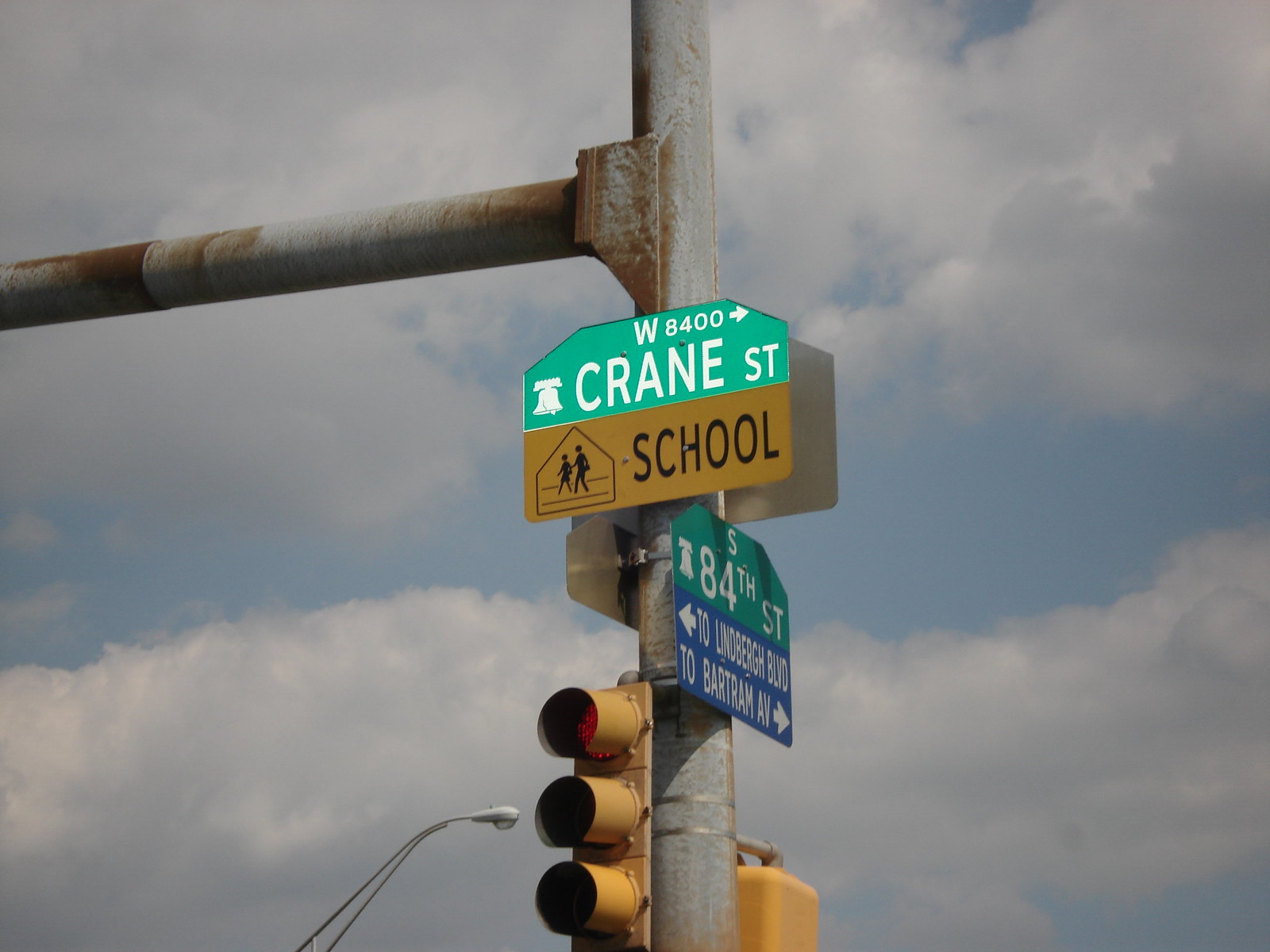This color photograph captures a street sign affixed to a pole, set against a backdrop of a blue sky punctuated by grey clouds. The lighting on the street sign notably contrasts the rest of the scene; the top of the sign is brightly illuminated and sharply in focus, while the lower section and surrounding elements appear dull and somewhat fuzzy, raising questions about photo manipulation or AI generation.

The central feature in the image is a tall, grey metal pole that extends vertically from the bottom to the top of the frame and then branches out horizontally towards the upper left corner. Several signs are attached to this pole. Prominently displayed is a green and yellow sign reading "W8400" in white text, accompanied by a right-hand arrow, a bell symbol, and references to "Crane Street."

Below this, a yellow sign with black text features the outline of a house and two walking figures, alongside the word "School." To the right of this sign, another sign appears with white writing, divided into a green upper section and a blue lower section, though its text is not legible in the image.

Beneath these signs, a set of traffic lights is faintly visible, with the red light seemingly dimly illuminated. Additionally, the edge of a streetlight is partially visible to the left of the traffic light, bearing a small, yellow protrusion to its right.